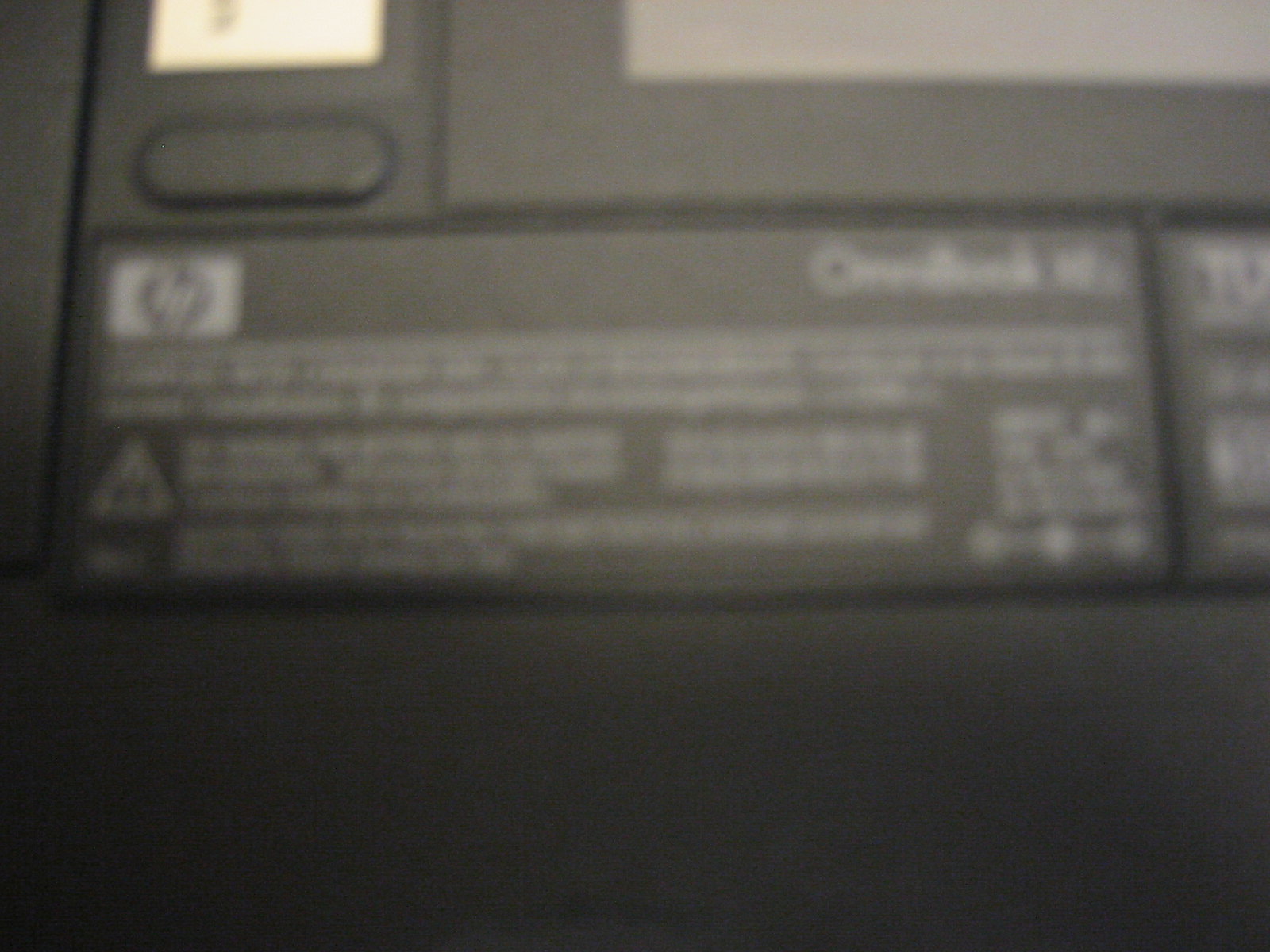The image depicts an extremely blurry, very zoomed-in close-up of what seems to be the backside of a laptop, particularly focusing on a battery compartment. The overall color scheme is predominantly dark gray or black. Central to the image is a rectangular area, which appears to be the battery, featuring an HP logo prominently on the left. Below the logo, there are lines of white text that are unreadable due to the blurriness. Above this section, there is a small foot or stand that the laptop would rest on when upright, and to the right of the battery is another section with a gray middle. Additionally, an oval gray button can be seen in the upper left corner of the image. The entire photograph is obscured by its excessive blurriness, making fine details indistinguishable.